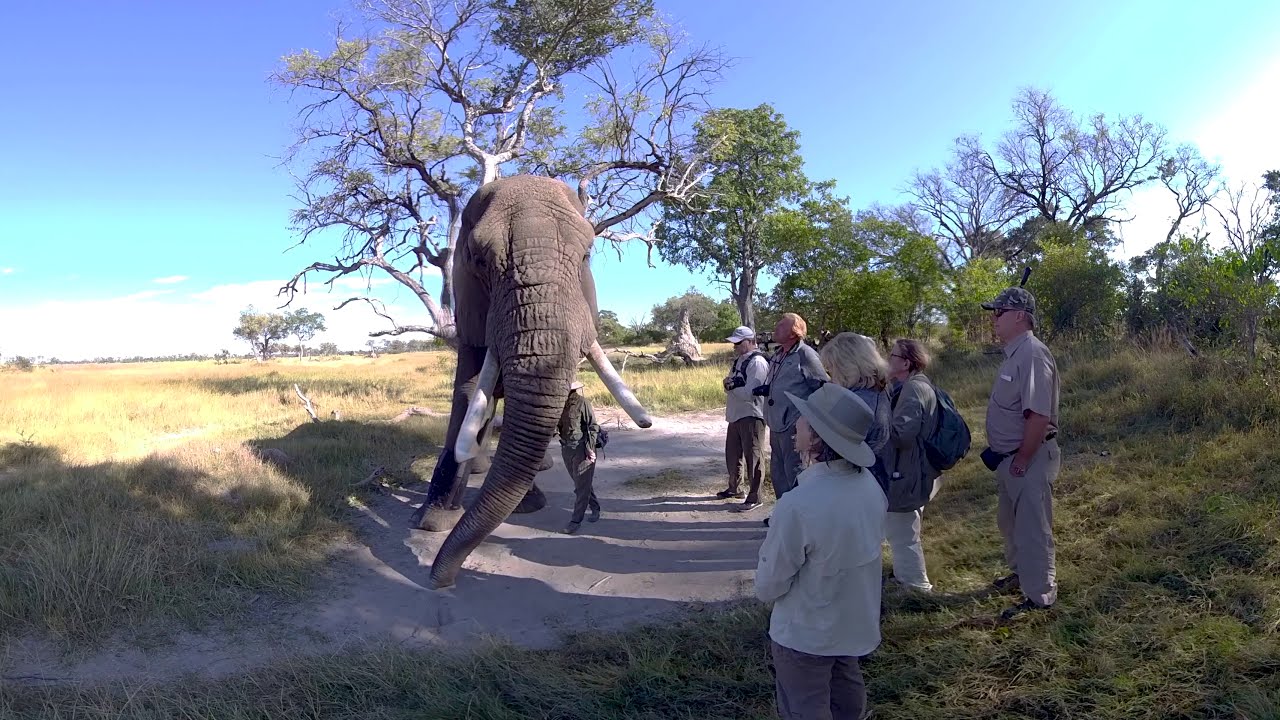The photograph, taken outdoors during a sunny day, presents a captivating scene set in a savannah-like landscape. At its center stands a large adult elephant, facing the camera, showcasing its gray trunk and large white tusks. The elephant dominates a dirt path that cuts through expansive, open grass fields—mostly composed of dry, yellow or brown grass, with patches of green interspersed. Sparse trees with varying amounts of foliage scatter across the background, contributing to the scene's serene yet wild nature.

Standing closely beside the elephant is a man, partially obscured by the elephant's trunk, seemingly interacting with or explaining the majestic creature. To the right of this central tableau, a group of at least half a dozen spectators observes the elephant with evident intrigue. Among them is a woman in a white jacket and gray hat, flanked by two other women, one of whom has long blonde hair. Noteworthy in the group are men with cameras around their necks: one dressed in blue, another in a white shirt paired with a baseball cap. A man in gray, also wearing a baseball cap and sunglasses, rounds out the assembly of onlookers.

The right side of the image is lush with greenery, more abundant in foliage and trees than the left, which features lighter, drier grass. The serene interaction between humans and nature captured in this photograph beautifully encapsulates the essence of an open, sunlit grassland.